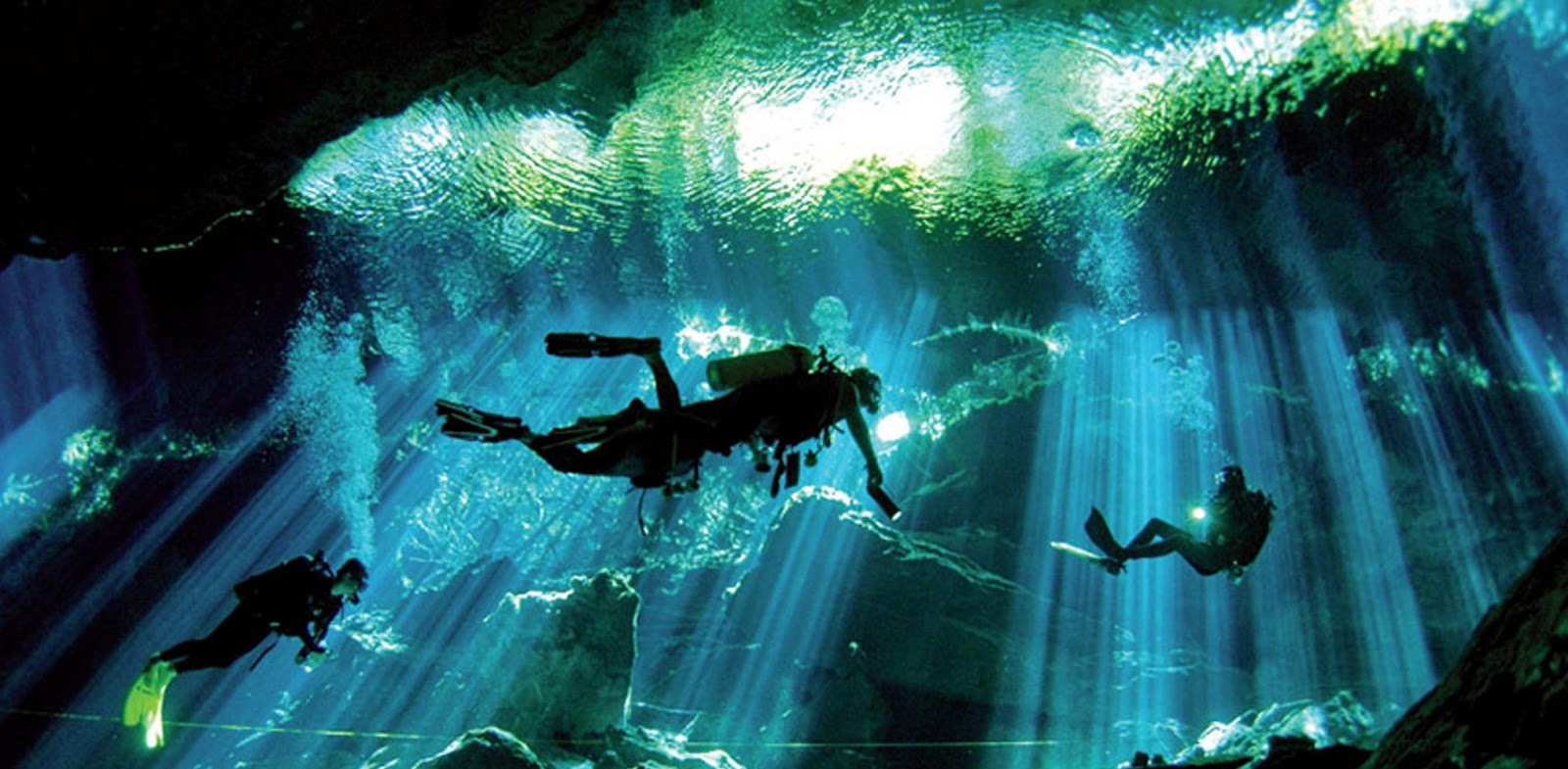An underwater photograph captures a mesmerizing scene of three scuba divers exploring an underwater cave. The image is taken from the bottom, looking up towards the surface where sunlight beams penetrate through the greenish-blue tinted water. The divers are silhouetted against the illuminated background, making their black wetsuits and oxygen tanks stand out. The diver to the left corner has bright yellow fins, while another in the middle has his arm extended forward holding a black flashlight. This diver is positioned horizontally, with his stomach facing the cave floor. To the right, a third diver appears to float in a seated position, also holding a flashlight. The rocky cave environment lacks much aquatic life, but some plants are visible. The divers create bubbles as they breathe, enhancing the dynamic underwater atmosphere, which blends darkness with the bright light from the sun above.